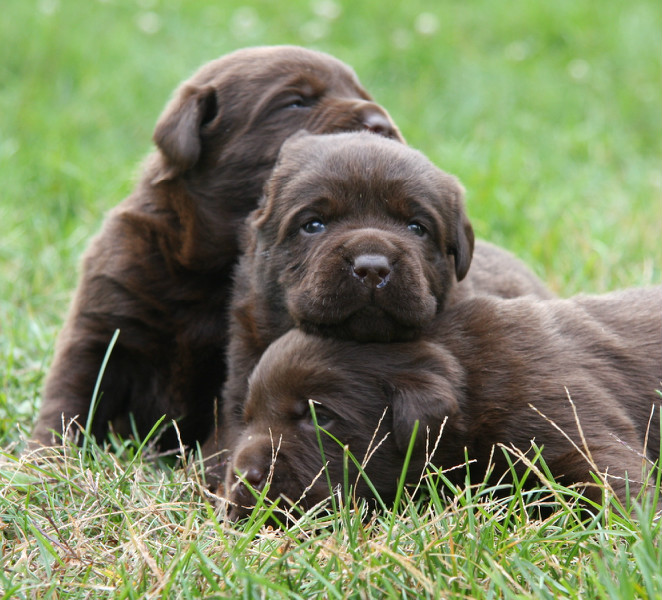In this outdoor daylight photograph, three chocolate brown puppies are peacefully resting in a field of vibrant green grass. The composition captures a tender and serene moment among the puppies, whose chocolate lab-like features include crinkled, floppy ears, brown noses, and deep brown eyes. The first puppy lies in the foreground with its head centered and torso extending to the right, gazing thoughtfully to the left. Resting adorably on its head, the second puppy is the focal point of the image, looking directly into the camera with a calm, sleepy expression. Just behind, the third puppy, partially obscured and peeking out from the left, gazes slightly off to his left towards the upper-right corner of the frame. The focused green grass in the foreground contrasts beautifully with the blurred background, emphasizing the tranquility and close bond of the tired, resting puppies.